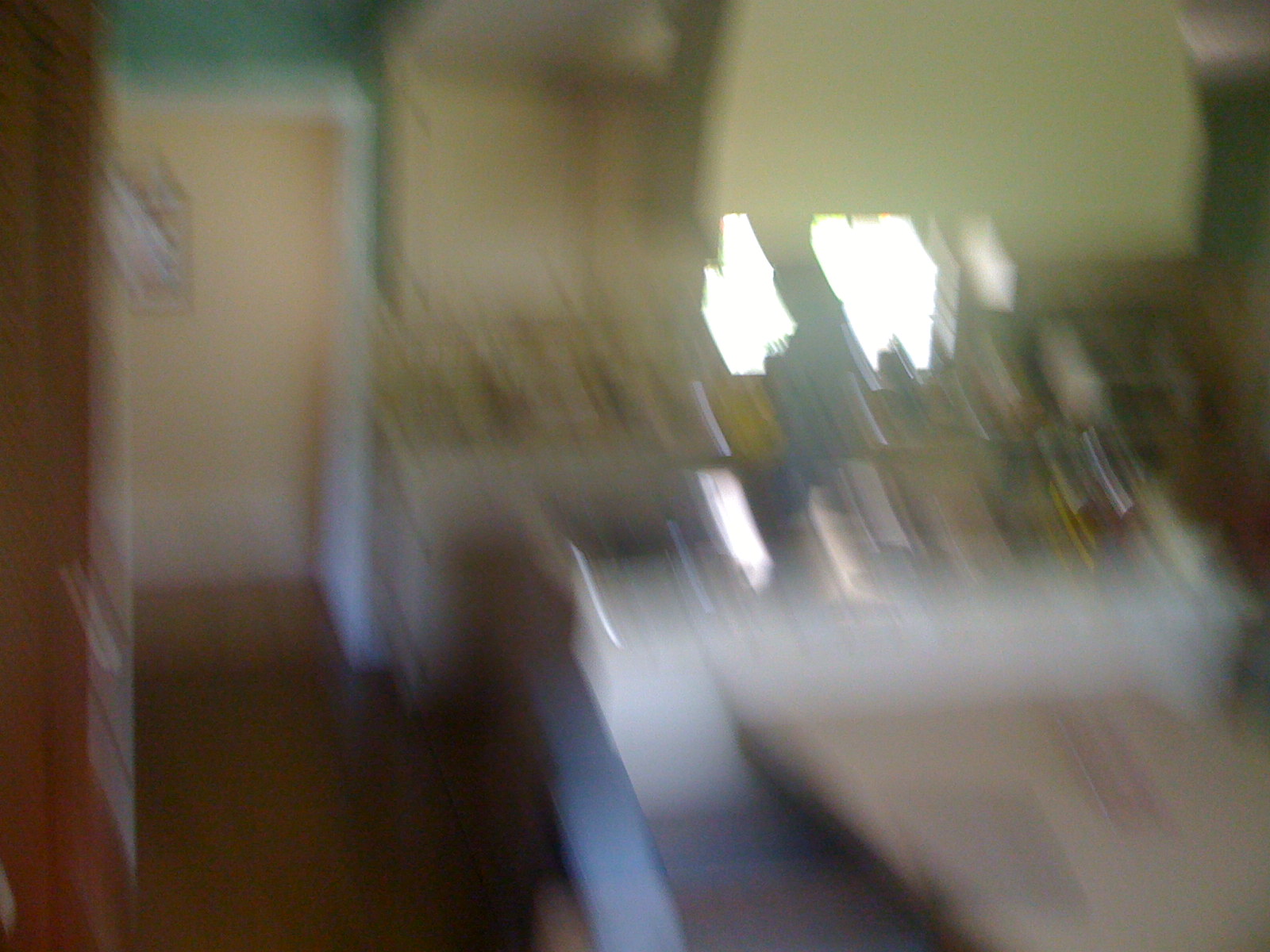In this extremely blurry photograph, seemingly taken inside someone's home, the outlines of various elements are faintly discernible. In the upper left corner, a large rectangular doorway is outlined in white, with a yellow-hued area in its center, suggesting an illuminated hallway or room beyond. To the left of this doorway, there appears to be a white door, possibly ajar. Moving to the right in the image, there is what looks like a white cabinet, though its details are indistinct. In the top right corner, a yellowish semi-circular form is visible, though its purpose or identity is unclear. Central to the photograph is the diffuse, scattered reflection from a window, punctuated by a multitude of indistinct light spots, which adds to the overall haziness of the image.